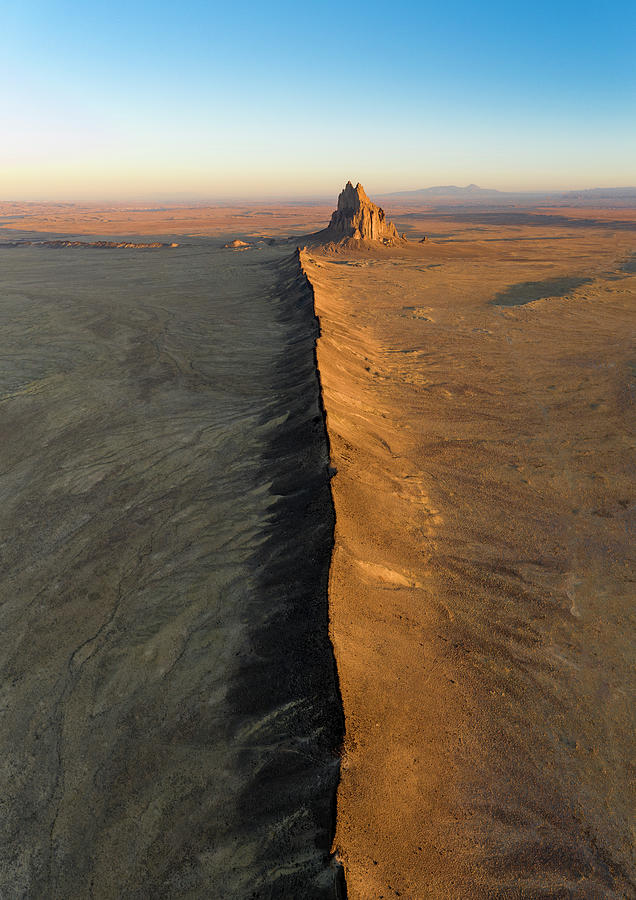This image captures a vast desert landscape dominated by a prominent mountain ridge that stretches vertically from the bottom center to about three-fourths up the photograph. The ridge is characterized by its sharp contours, with the right side brightly illuminated in an orangey-brown hue by sunlight coming from the right, while the left side remains in shadow, imbued in a dull tan-brown. The central ridge converges into a small craggy hill in the distance, beyond which lie additional low hills on the horizon. To the far right, a small body of water, possibly a lake or pond, contrasts with the arid surroundings. The sky above occupies roughly a quarter of the image, transitioning from a dark blue near the top to a whitish-blue and then a subtle yellow closer to the ground. This composition highlights the stark beauty and varied texture of the desert terrain, split between sunlit and shadowed expanses, with every element bathed in a palette of sandy reds, pale whites, and earthy browns.